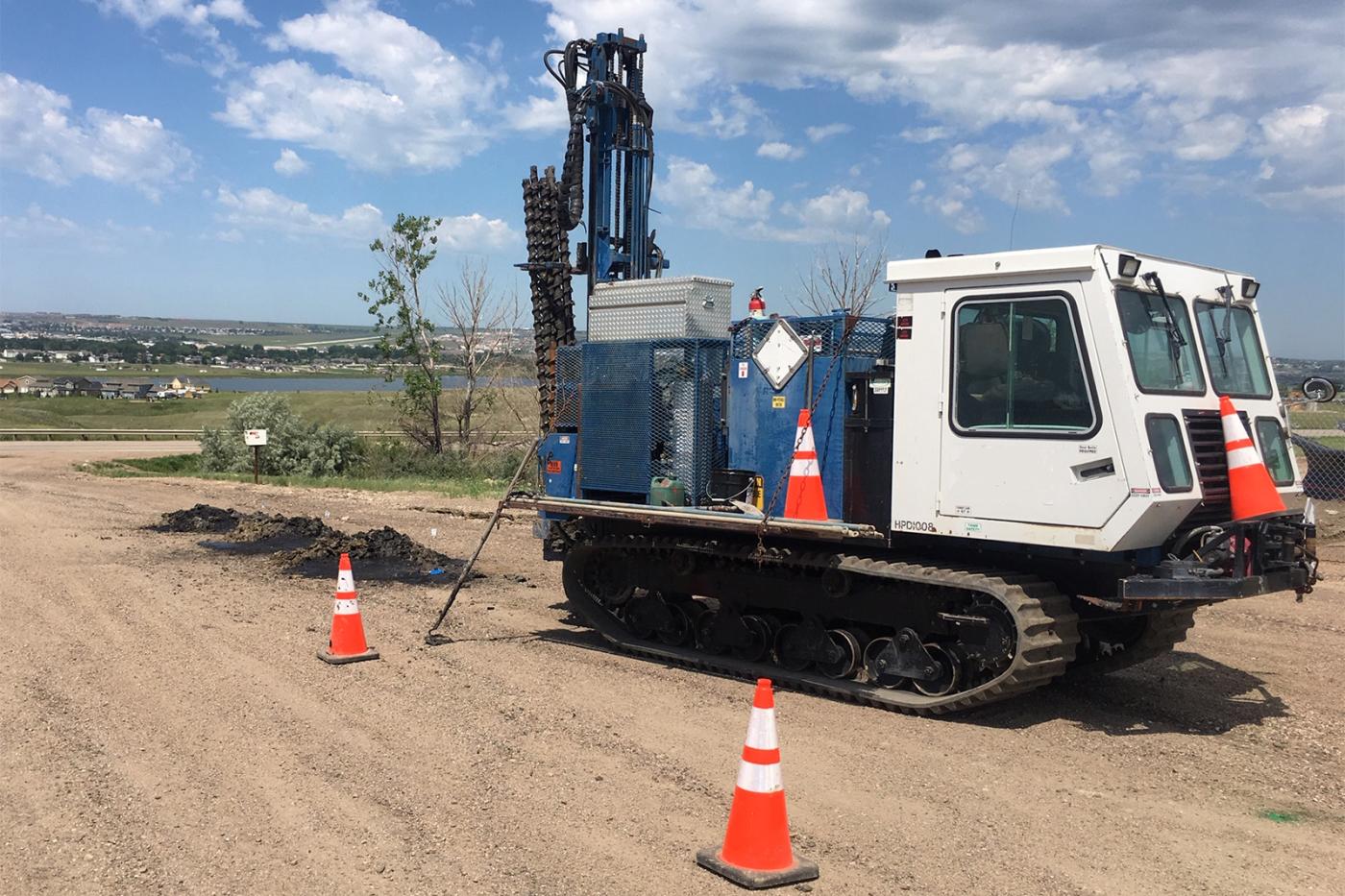This photograph depicts a construction site on a dirt road, featuring a robust piece of heavy equipment. The vehicle, which boasts a white, boxy cab, is equipped with rubber tracks that provide its tank-like propulsion. Behind the cab, the flatbed holds a complex arrangement of blue and silver boxes, possibly containing flammable fluids such as propane or diesel fuel. Prominently visible are an orange traffic cone on the front and another on the side of the vehicle, as well as two additional cones positioned nearby to demarcate the work area. A metal pole with attached chains rises from the back, indicating that this vehicle is likely used for drilling or ditch digging. There is also a hose draped along the side. Behind the equipment are three small piles of disturbed black dirt, suggesting recent digging activity. The background showcases a picturesque scene with a blue sky dotted with white, puffy clouds, a residential area with houses and trees, and a large lake or body of water, adding a serene contrast to the industrious foreground.